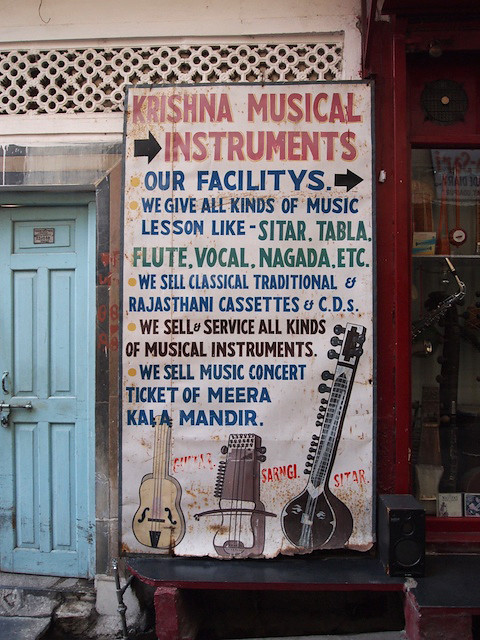The scene depicts a large, old, and slightly dilapidated sign affixed to a wall. The sign, which has seen better days, reads "Krishna Musical Instruments" at the top in bold red letters and includes an arrow pointing to the right, indicating a storefront. The text on the sign provides detailed information about the store's offerings: "Our Facilities. We give all kinds of music lessons like sitar, tabla, flute, vocal, nagada, etc. We sell classical, traditional, and Rajasthani cassettes and CDs. We sell and service all kinds of musical instruments. We sell concert tickets of Meera, Kai, and Mandir." Below the text, there are illustrations of various musical instruments, including a long-neck sitar. To the left of the sign is a light blue door, partially framed by a cement stoop. To the right of the sign, within the storefront window, is a display case showcasing an array of musical instruments. A speaker is positioned at the bottom right near the stand, completing the scene with an array of colors including red, white, faded red, blues, greens, browns, blacks, beige, baby blue, and burgundy.